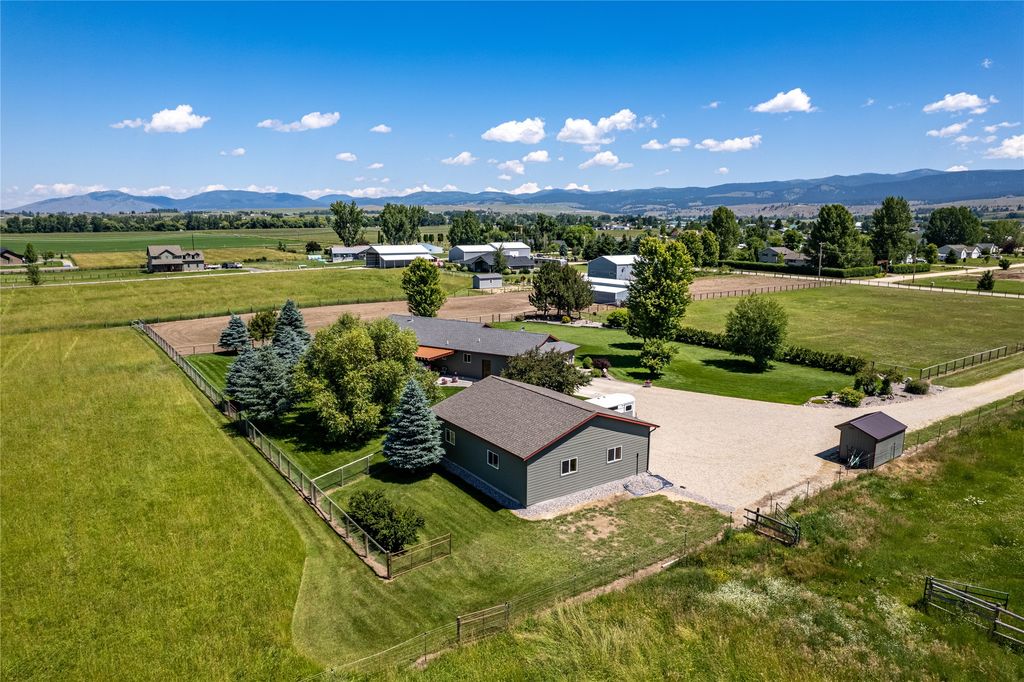This aerial photograph, likely taken with a drone, showcases an expansive rural or agricultural property, probably a horse ranch. Dominating the foreground is a house accompanied by an outbuilding, possibly a garage with a horse trailer parked in front. Adjacent to the garage are stable-like structures, suggesting areas designated for horse care and training. The property is lush with vibrant green grass, indicative of the summer season, and dotted with various trees, including green and blue spruce. 

The property spans a wide area, surrounded by fences that define the boundaries. Multiple buildings scattered across the property likely serve different functions, from housing to storage. A long driveway meanders through the scene, lined with green lawns. The background reveals additional houses and outbuildings, giving a sense of a larger neighborhood or ranch compound. 

Far in the distance, the view extends to a majestic mountain range under a wide blue sky mottled with white clouds, hinting at the beauty and expanse of the surrounding landscape. This detailed scene embodies a picturesque, well-maintained rural horse ranch, blending living areas seamlessly with functional spaces for horse breeding and care.